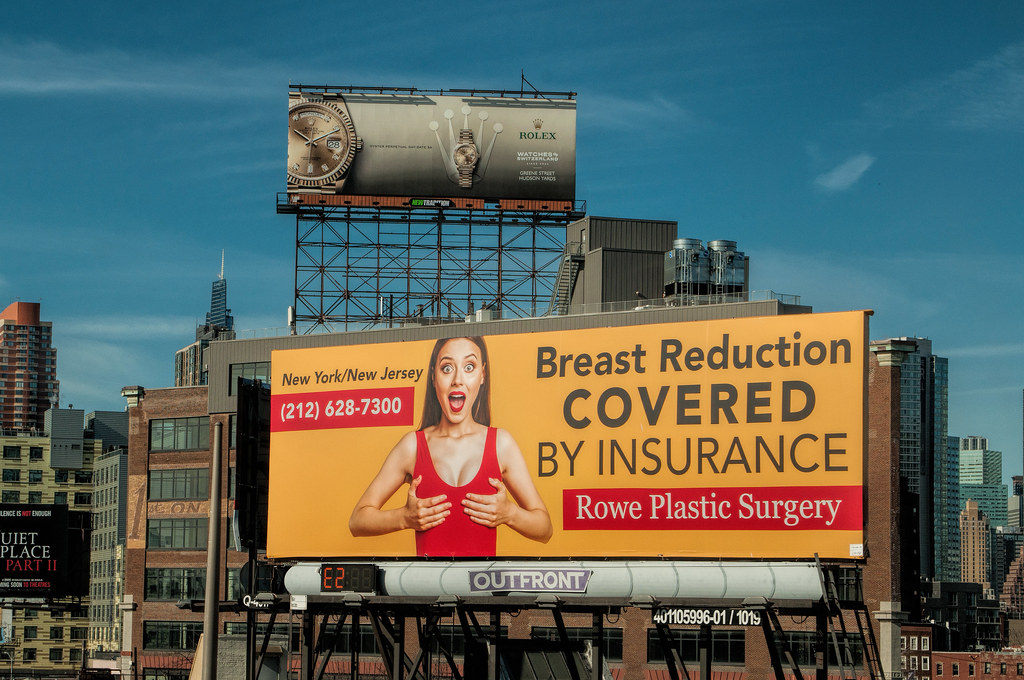This image captures a prominent billboard located atop a rooftop, with the camera positioned at the same elevation as the billboard. The billboard itself is a dark yellow color, featuring black text that reads "New York / New Jersey" and "brush reduction covered by insurance." Additionally, in white letters on a red banner, it advertises "rope plastic surgery." The advertisement includes a photograph of a woman wearing a tank top, posing with a cheerful expression, her mouth open, and her hands placed on her breasts.

In the background, the urban landscape is visible with numerous buildings stretching out behind the primary billboard. One of these buildings hosts another billboard, which is gray and displays an image of a watch. The sky above is a clear blue, adorned with several wispy clouds adding a subtle texture to the scene.